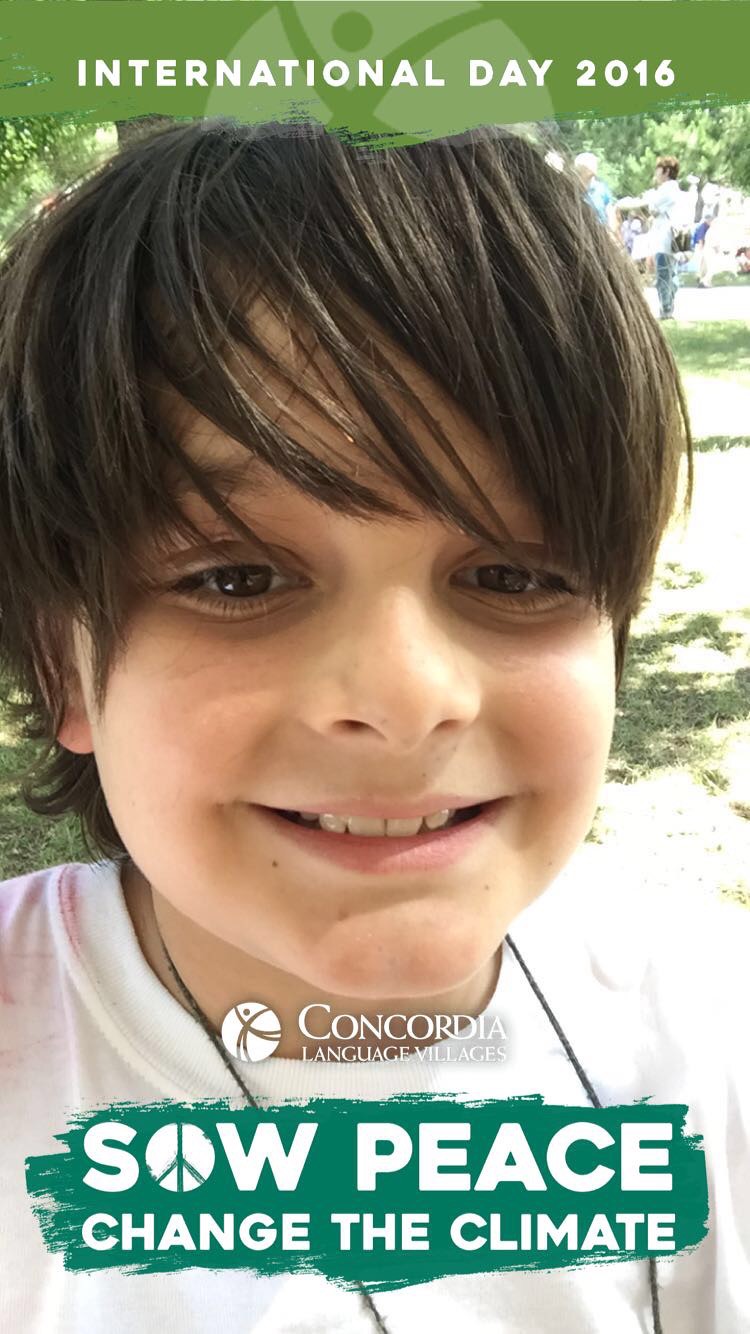The image is a vibrant outdoor scene capturing a young Caucasian boy with a joyous smile, clearly at ease. He is close to the camera, allowing a detailed view of his long, shaggy brown hair that is gently swept to the side of his forehead. His expressive brown eyes and the light pink of his smiling lips add warmth to the overall composition. The boy is dressed in a simple white T-shirt at the center of which lies a green scribbly line background with white text reading, “So SOW Peace Change the Climate” where the "O" is replaced by a peace sign. Around his neck is a black necklace, partially obscured, with the lower portion cut off by the bottom edge of the photo. The backdrop is rich with trees, foliage, and hints of a grassy field, suggesting it's a sunny day with clear blue skies accentuated by the presence of shadows. Additional hints of people, possibly adults, are visible at the top right corner of the image. A green horizontal bar at the top with white text announces "International Day 2016," and at the bottom, the logo of Concordia Language Villages is visible, establishing the context of the event. The scene is an energetic celebration of international unity and peace.